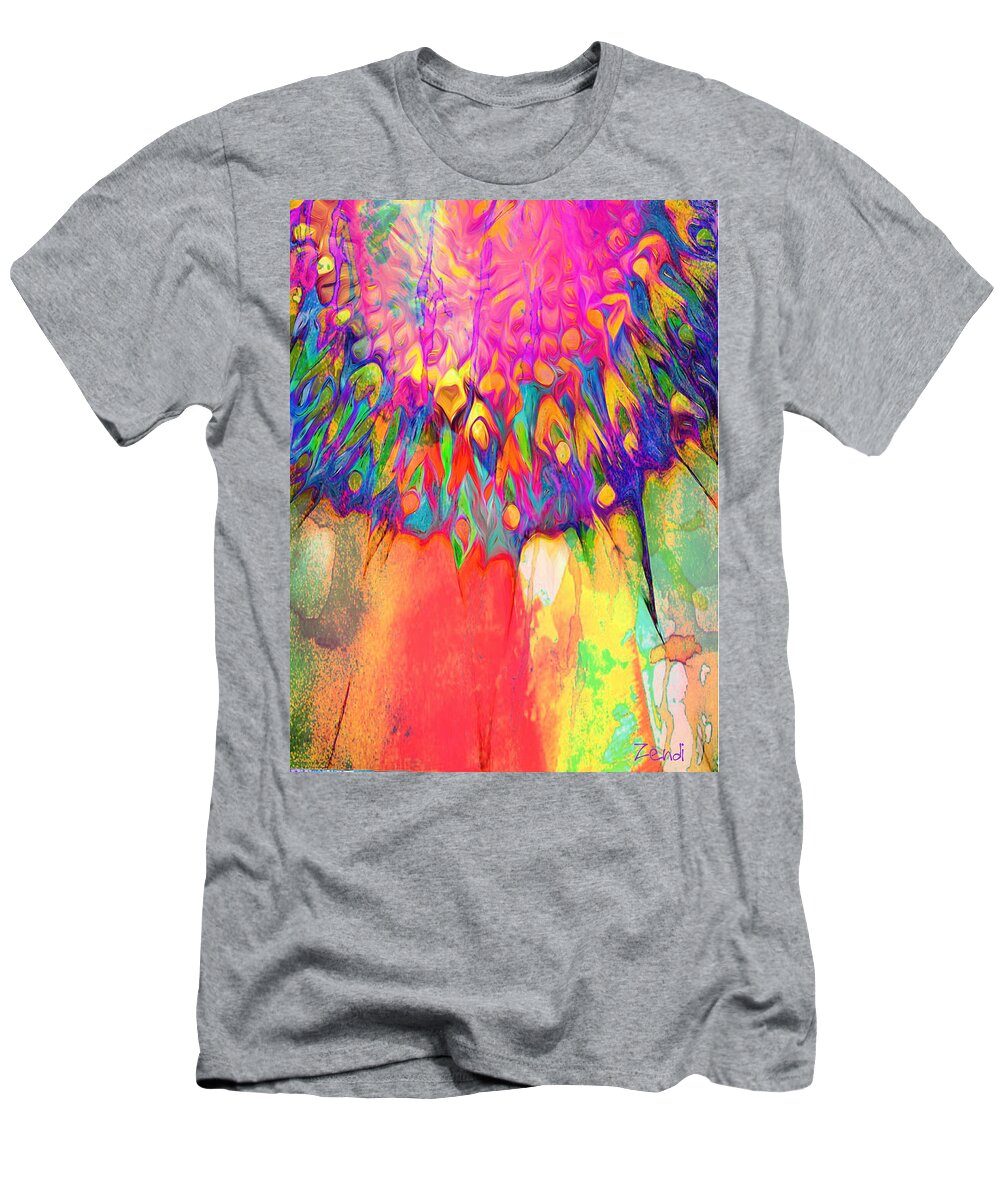This image features a plain gray crew neck t-shirt with basic sleeves, set against a bright white background. The t-shirt appears slightly wrinkled and prominently displays a large square design starting just below the collar. The design within the square showcases an array of vivid, neon-like colors including bright pink, lime green, orange, yellow, blue, and teal. These colors appear almost psychedelic and seem to be melting or smearing downwards, reminiscent of a tie-dye effect but on paper. The vibrant hues create a stark contrast against the muted gray fabric, making the design pop. Despite the intricate artwork, there is no text or writing present in the image. The overall impression suggests that the design may be a separate piece lying on top of the t-shirt, perhaps photoshopped to visualize the final product for potential customers.